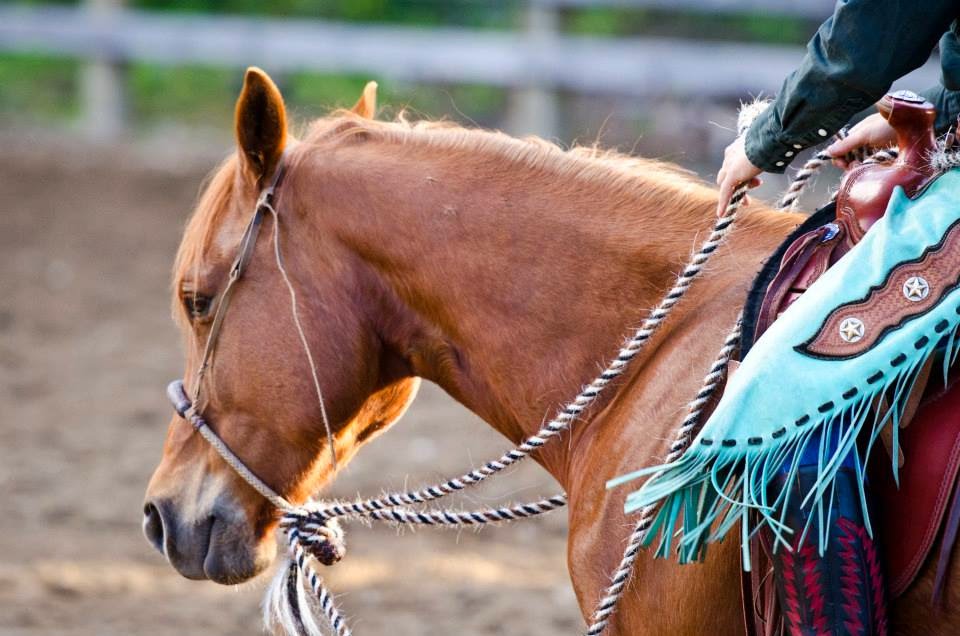The color photograph depicts a scene of horseback riding, capturing the lower body and hands of the rider and the head and upper body of the horse. The horse is a light brown color with a distinctive short blonde mane that extends over its forehead, partially covering its eyes. It also has a black nose and mouth. The rider, positioned to the right side of the photograph, is outfitted in black and red tooled leather cowboy boots, turquoise chaps with aqua fringe, and a decorative two-star pattern. They also wear jeans and a long-sleeved shirt with a button cuff. The rider’s hands are gripping braided reins made of white, brown, and blue fibers, which are attached to a simple halter around the horse’s muzzle, forgoing a traditional bridle and bit. The western-style saddle features a tall pommel and complements the rider's western attire. The backdrop includes a blurred wooden split-rail fence and lush green foliage, indicating the setting is a paddock or horse track.